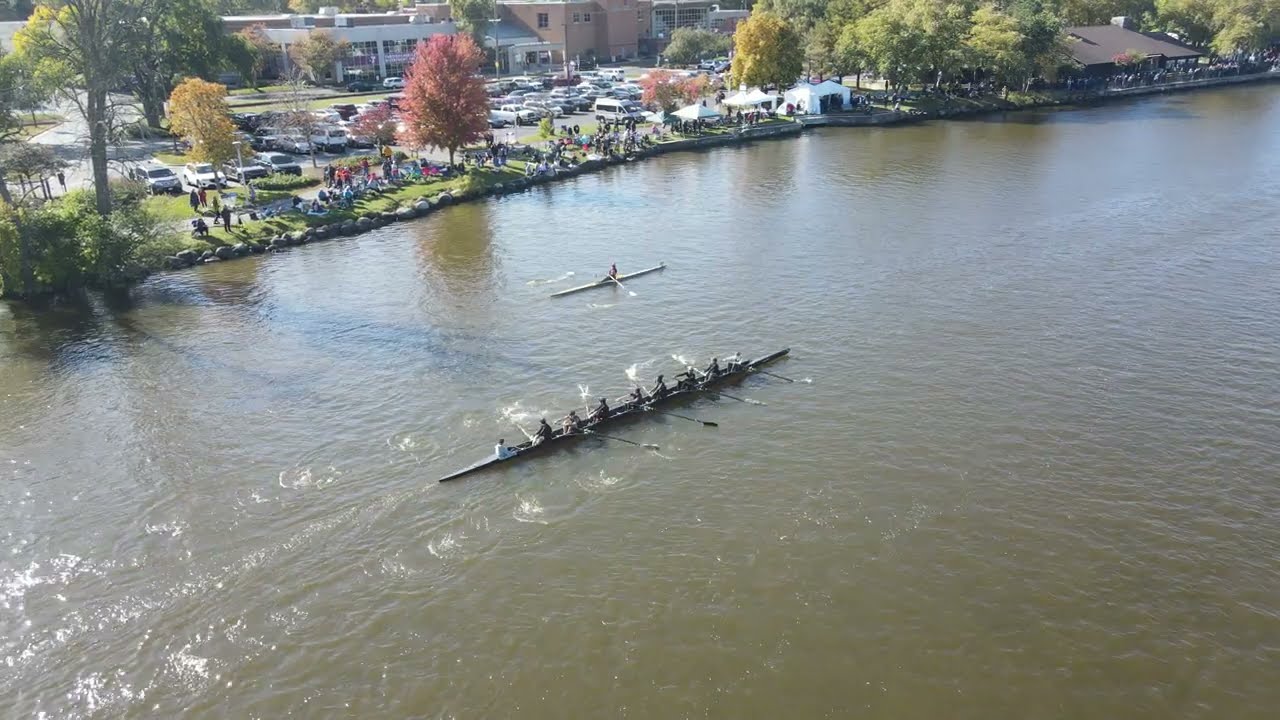This aerial photograph captures a dynamic scene of a rowing competition on a wide, murky brown river. At the center of the image, a sleek, long rowing boat with eight rowers and an instructor, known as a coxswain, who is urging them to row, glides through the water. The rowers are strategically positioned to paddle with long oars on either side, demonstrating synchronized movement. Adjacent to this boat is a smaller, one-person rowing boat, often referred to as a scull, with a rower paddling steadily, likely not part of the race.

The river occupies the majority of the lower and right areas of the photograph, while the left side showcases a grassy bank teeming with spectators. These onlookers are gathered along the edge, tents indicating areas probably set up for refreshments or event accessories. Behind them, a large parking lot congested with cars is visible, suggesting a significant turnout. The backdrop includes a few industrial or office buildings, hinting at an urban environment. Scattered among this setting are various trees, some displaying vibrant green foliage, while others show hues of red and yellow, indicating the onset of fall.